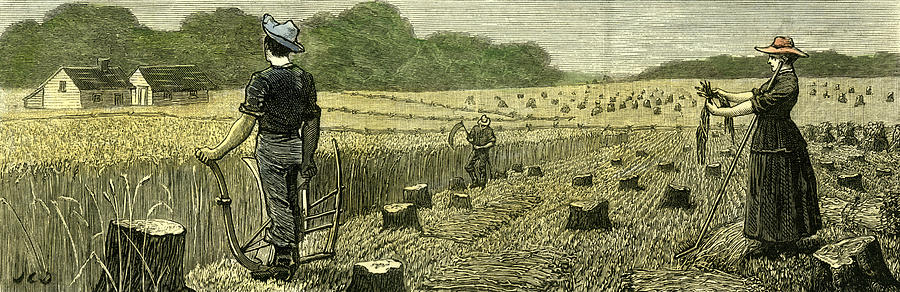The image depicts a detailed old-school style drawing of three people laboring in a field of wheat or hay, with some bundles already tied up. On the left side of the drawing, there are two simple houses situated next to each other, with a dense gathering of trees and bushes in the background. The field is scattered with tree stumps, suggesting recent clearing. On the right, a woman in a long dress with her sleeves pushed up and wearing a red hat is tying together bundles of wheat. She has a rake either leaned against her or in her hand. In the middle, a man with a hat is gazing downward while carrying a scythe. To the left, another man in a blue hat holds a tool, possibly looking towards the houses. The scene is serene yet bustling with the diligent activity of farm laborers.